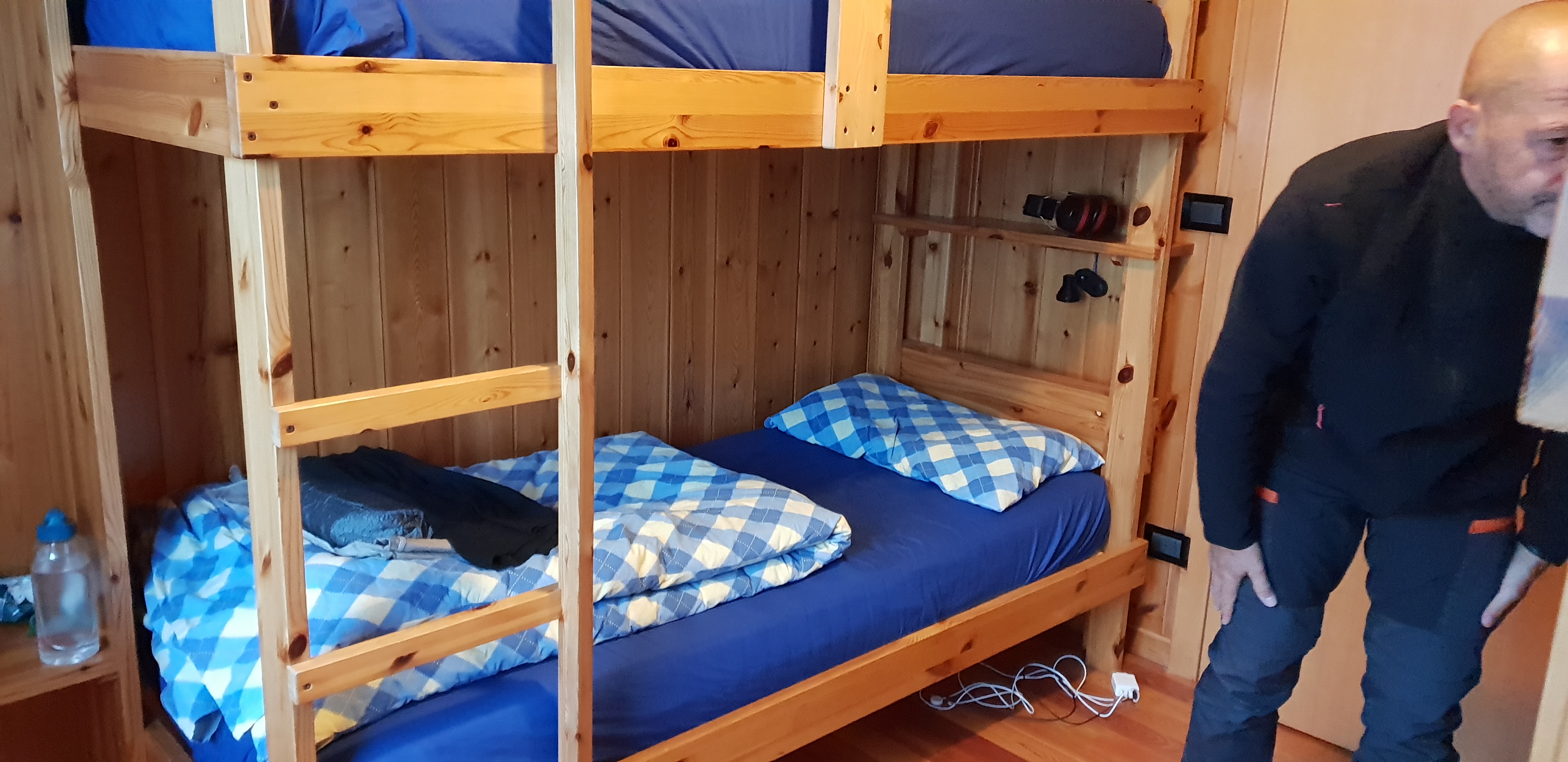The photograph depicts a cozy cabin bedroom with pine wood-paneled walls and hardwood floors. On the left side of the image, there is a set of light-colored wooden bunk beds, positioned at a slight diagonal toward the one o’clock direction, pushed into a corner where the wall division is roughly 60% from the left. The bunk beds feature dark blue mattress covers, with the bottom bunk additionally adorned with neatly folded white and light blue checkered blankets and pillowcases. Under the bunk bed, a white phone charger cable is visible on the floor. Adjacent to the bed, on a shelf, there is a water bottle with a blue top.

On the right side of the image, a bald man with a fair complexion, partially visible due to the framing of the photo, is standing and facing right. He is dressed in a black long-sleeved shirt and blue pants with notable orange zippers on the pockets. The intricate details and rustic charm of the cabin bedroom, combined with the presence of the individual, paint a serene and detailed scene of simple, comfortable living.